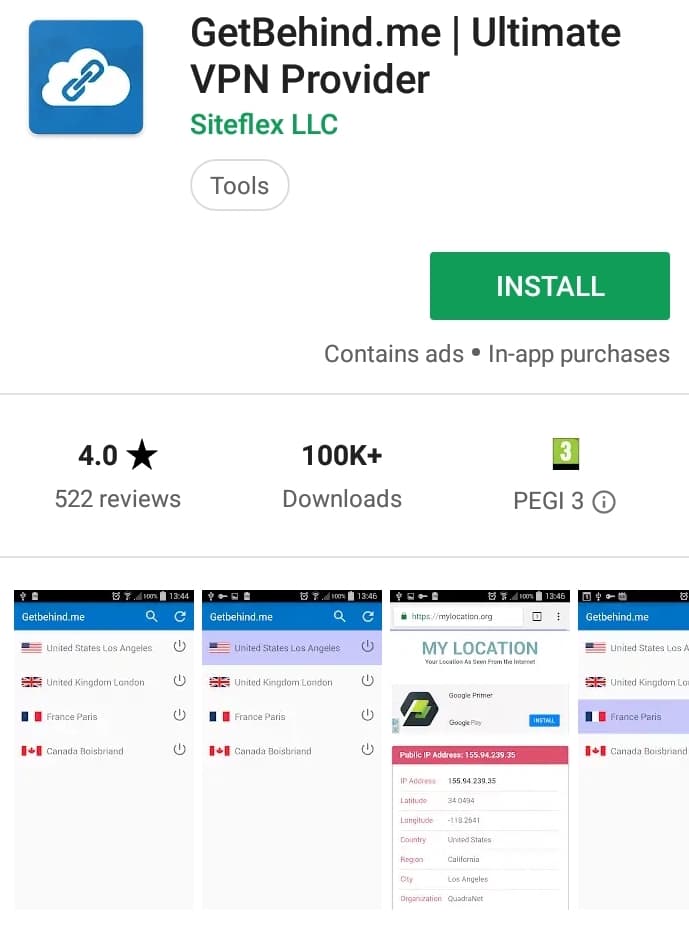The image depicts a selection screen from either the Google Play Store or the Apple App Store, showcasing the app “getbehindme.me.” The layout is in portrait mode on a solid white background with no border. In the upper left corner is the app icon, a blue square featuring a cloud with a small chain inside of it. The app's name is “getbehindme.me,” followed by a subtitle, “Ultimate VPN Provider.” The developer, Siteflex LLC, is then mentioned. Below that, a tag states that this is a tool.

To the right and just below this information is a prominent green “Install” button. Below this button, details about the app indicate that it contains ads and offers in-app purchases. Further down, there is a row with information on user reviews, number of downloads, and the app's PEGI rating of 3. 

A thin gray line separates this section from a series of four screenshots, which display the “getbehindme.me” app in action. The screenshots showcase various features of the app, such as country settings and operational views, laid out side by side across the screen.